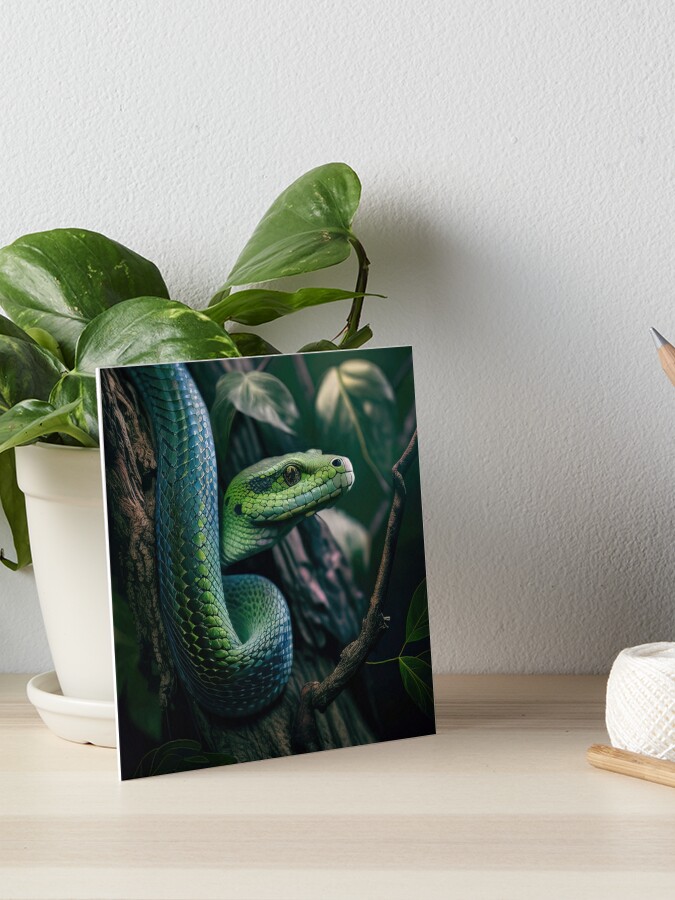The photograph captures a serene, intimate scene in what appears to be a cozy room. On a desk made of light beige wood with distinct horizontal stripes, a stylized painting of a snake is prominently displayed. This intricate artwork depicts a green and blue-scaled snake coiled around a dark brown tree trunk, with its head peeking out just above the center of the frame, looking to the right. Green leaves embellish the top and bottom right corners of the painting, adding a touch of natural beauty. The painting leans against a pristine white flower pot with a matching white saucer, from which broad green leaves sprout energetically. To the right of the composition, a twisted ball of white yarn partially exits the frame, sitting next to a small piece of wood. Above this, the very tip of a pencil, its gray graphite and wooden body truncated by the frame's edge, subtly peeks into view. The background is a smooth, mottled white wall, casting gentle shadows that add depth and dimension to the tranquil setting.